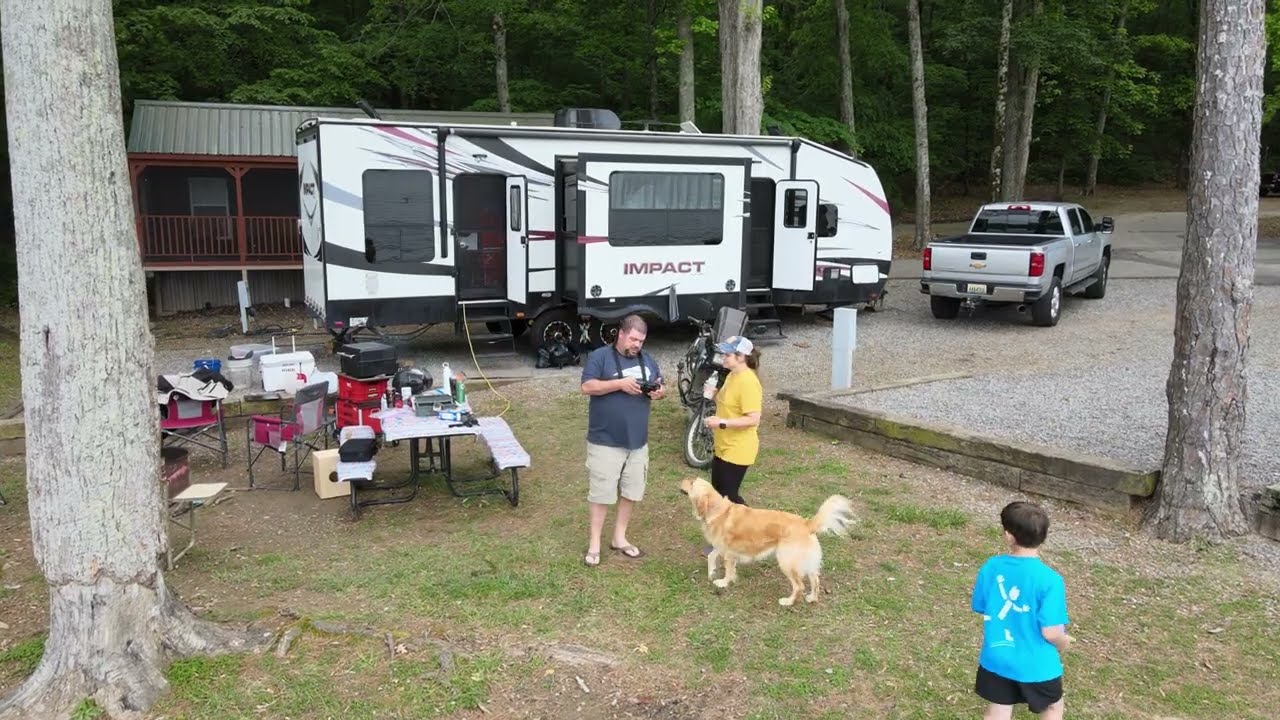This photo captures a campsite scene where three people and a dog gather in front of a large white and yellow RV labeled "Impact," set against a backdrop of a modest lodge-like cabin. The RV is parked next to a silver pickup truck in a wooded area with an array of green-leafed trees and a gravel parking space. The grass in the foreground appears worn, flanked by two large tree trunks.

In the center, a man in a navy blue shirt and cargo shorts stands examining his camera, drawing the attention of a woman in black pants and a yellow t-shirt, a golden retriever wagging its tail, and a child in black shorts and a light turquoise blue shirt. The cluttered picnic tables nearby are strewn with various items, possibly including a red portable grill with a black top. Additional camp chairs are set around the area, adding to the disorganized yet cozy campsite vibe.